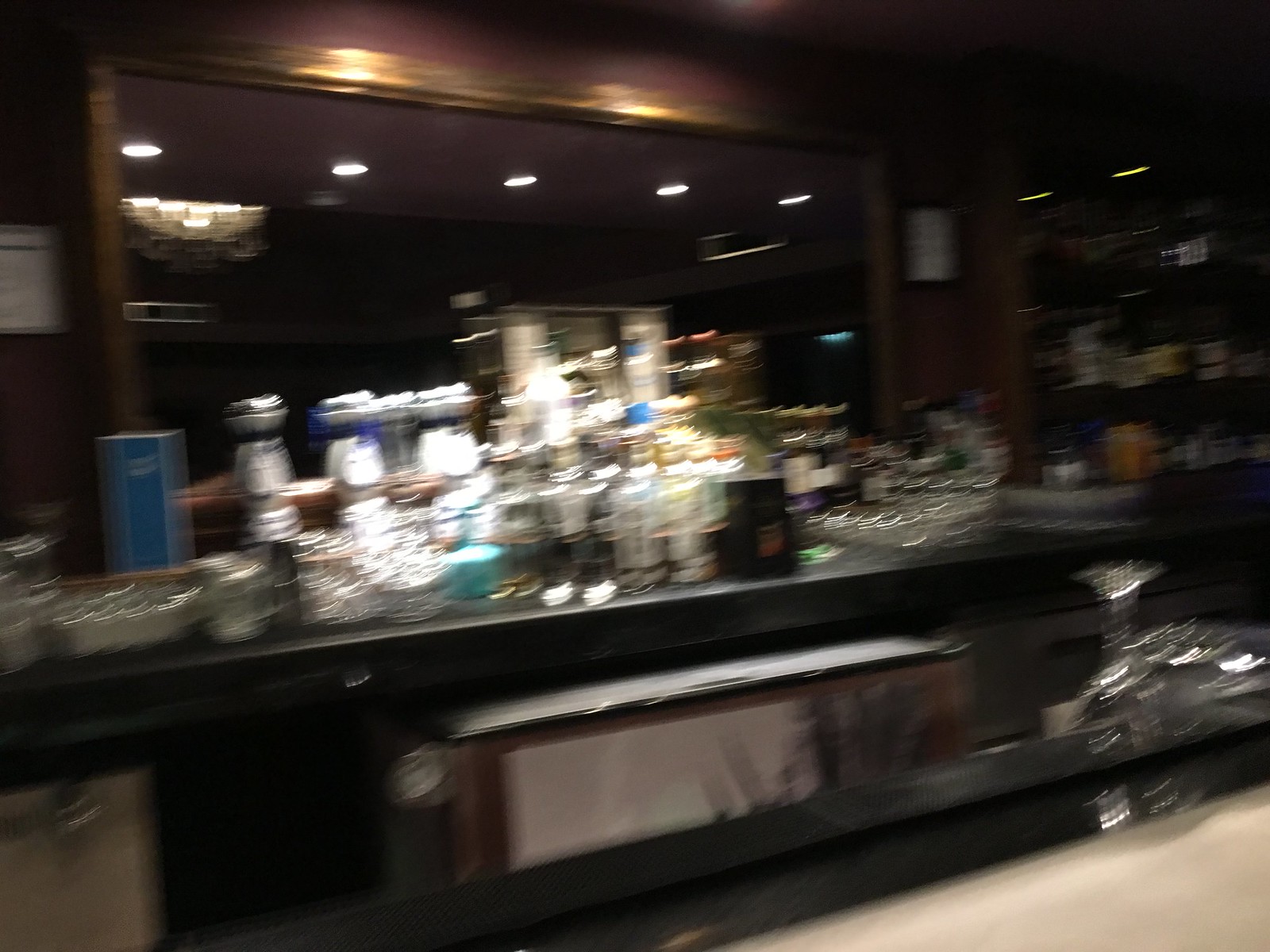In the center of the room stands an island bar with a sleek, chrome, shiny countertop. The bar is adorned with an array of glass bottles, showcasing a variety of colors and adorned with diverse stickers. Overhead, small lights illuminate the scene, casting a soft glow on the glass bottles. Flanked on both the right and left sides of the bar are neatly arranged clear glasses. In the background, a plaque hangs on the wall, underneath a ceiling studded with round lights. On the wall to the right, several white square decor pieces add a modern touch. Additional clear cups are positioned in the front right corner of the bar, completing this chic and contemporary setting.